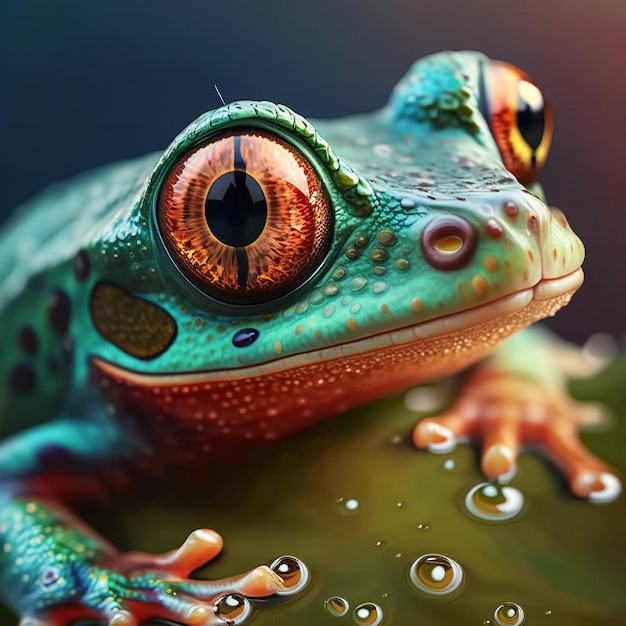The image is an extremely detailed, close-up portrayal of a tree frog, vivid and intricate enough that it might be mistaken for a highly skilled painting or a digital creation. The photograph captures the entirety of the frog within a dark background, highlighting its dominating presence. Its large, almost golden eyes with black pupils seem to gaze directly at the viewer, exuding a striking presence.

The frog's skin is a kaleidoscope of colors and patterns. The top of its body is predominantly green with teal and brown dots, transitioning into an array of intermingled orange, red, and amber shades as you move down its body. The nostrils are crimson, adding a deeper hue to its detailed features, while the top of the mouth is light green adorned with orange and red circles. The underside of the mouth and the frog’s belly is a gradient of orange, ranging from light to a darker reddish-orange.

Its front legs are positioned in the water, with visible bubbles enhancing the sense of realism and bringing texture to the scene. The legs themselves are teal on top, transitioning to orange underneath, with particularly prominent orange coloring on its webbed fingers. A fascinating detail is the tiny black speck under the frog's eyes and a single hair strand sticking out from the top of its left eyelid, adding both authenticity and a slightly whimsical touch.